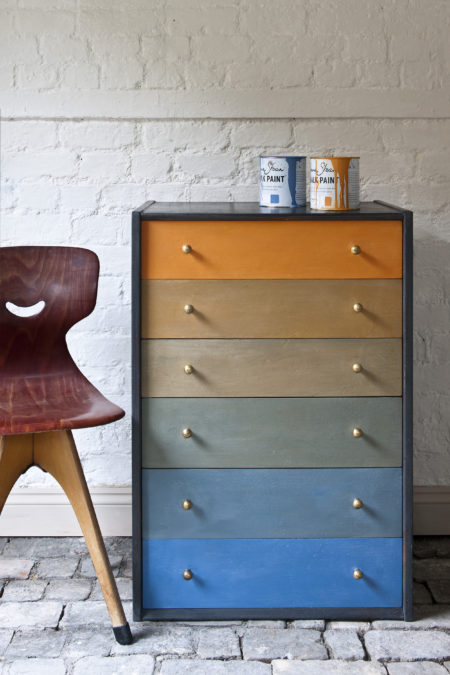The image showcases a tastefully renovated chest of drawers, set against a white-painted brick wall with a gray paver stone floor. The chest, with a black exterior and six differently colored drawers, stands about chest-height. The drawers, from top to bottom, are painted in vibrant hues: orange, orangish brown, brown, bluish brown, light blue, and bright blue. Each drawer features two elegant golden knobs. On top of the chest, a blue and an orange paint can rest, with paint visibly dripping down their sides, hinting at an artistic touch. To the left of the chest, a portion of a sleek, modern wooden chair is visible. The chair has a curved dark brown silhouette with a small, smiley-face-like cutout in the center and sturdy thick prongs at the base. The scene is both rustic and contemporary, highlighted by the detailed textures of brick and stone, and the vibrant, yet harmonious, color scheme of the furniture.